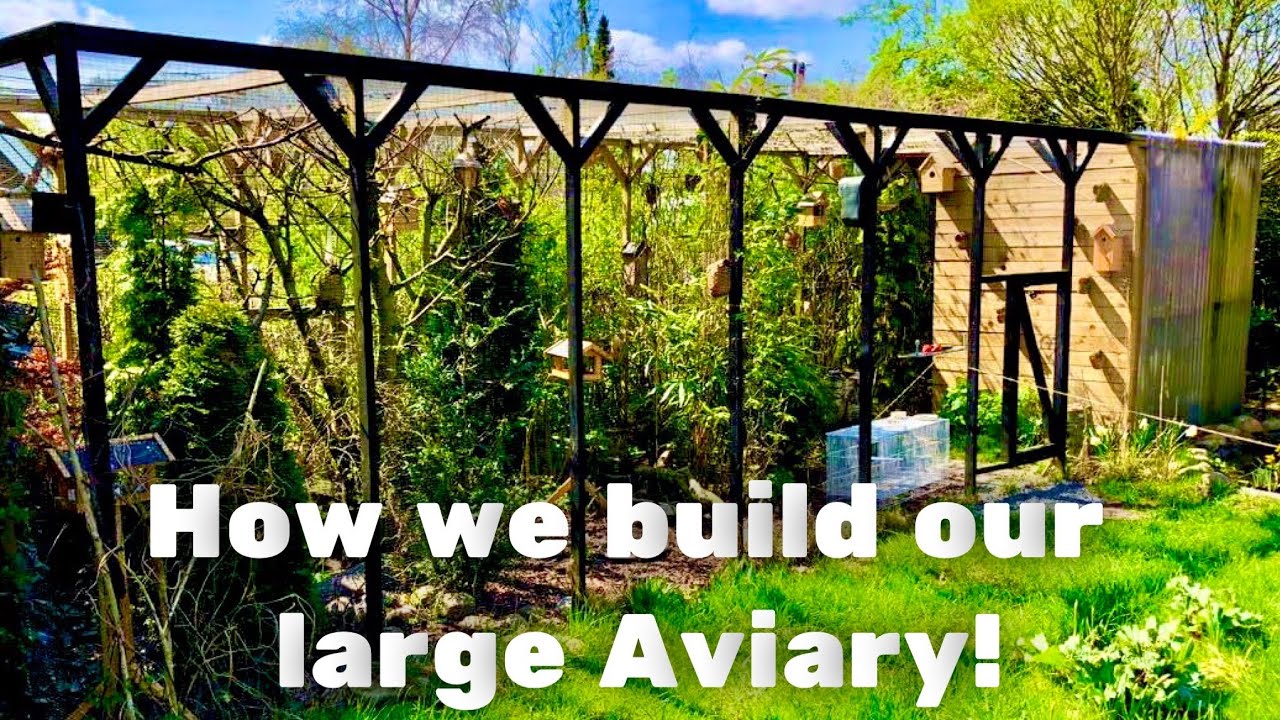This outdoor photograph showcases a partially constructed aviary within a backyard setting. Dominating the image is a black wood frame structure, which appears to serve as the primary framework for the aviary, accompanied by some fencing that is difficult to discern. Inside the enclosure, we can see an abundance of trees, bushes, and various plants. Scattered throughout the greenery are small, hard-to-spot birds. To the right of the aviary structure, there is a well-maintained green lawn, extending up the side of the image. The scene is bathed in sunlight, with blue sky and white clouds visible through the foliage above. Large white text overlays the bottom of the picture, reading "How We Build Our Large Aviary!" The text accentuates the ongoing construction and hints at the future role of the enclosure in housing birds.